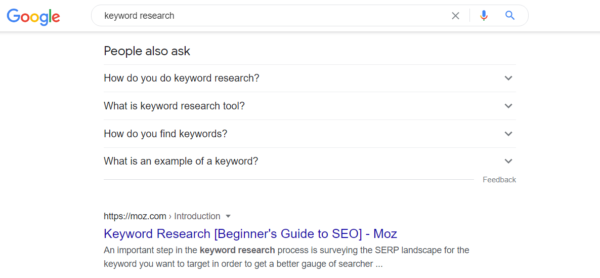This image is a screenshot of a Google search results page with an all-white background. Prominently displayed in the upper left corner is the multicolored Google logo. Adjacent to the right is an oval-shaped search bar containing the text "Keyword Search" in black lettering. To the far right within the search bar are a gray "X," a multicolored microphone icon, and a blue magnifying glass icon, representing the voice search and search functions respectively.

Beneath the search bar, a horizontal gray line spans the width of the screen. Directly under this line is a section labeled "People Also Ask" in black text. This section includes a series of concise questions related to keyword searches, each followed by a down arrow on the right to expand for more information:
1. "How do you do keyword search?" - Down arrow
2. "What is Keyword Research Tool?" - Down arrow
3. "How do you find keywords?" - Down arrow
4. "What is an example of a keyword?" - Down arrow

At the bottom of this list, the word "Feedback" appears in light gray text, with another horizontal gray line to the left of it.

Below the "People Also Ask" section is a search result for "moz.com," with an introductory snippet indicated by a down arrow. The result features a prominent, bold, large, blue header that reads "Keyword Research [Beginner's Guide to SEO-MOZ]." The description underneath states, "An important step in the keyword research process is surveying the SERP landscape for the keyword you want to target in order to get a better gauge of searches."